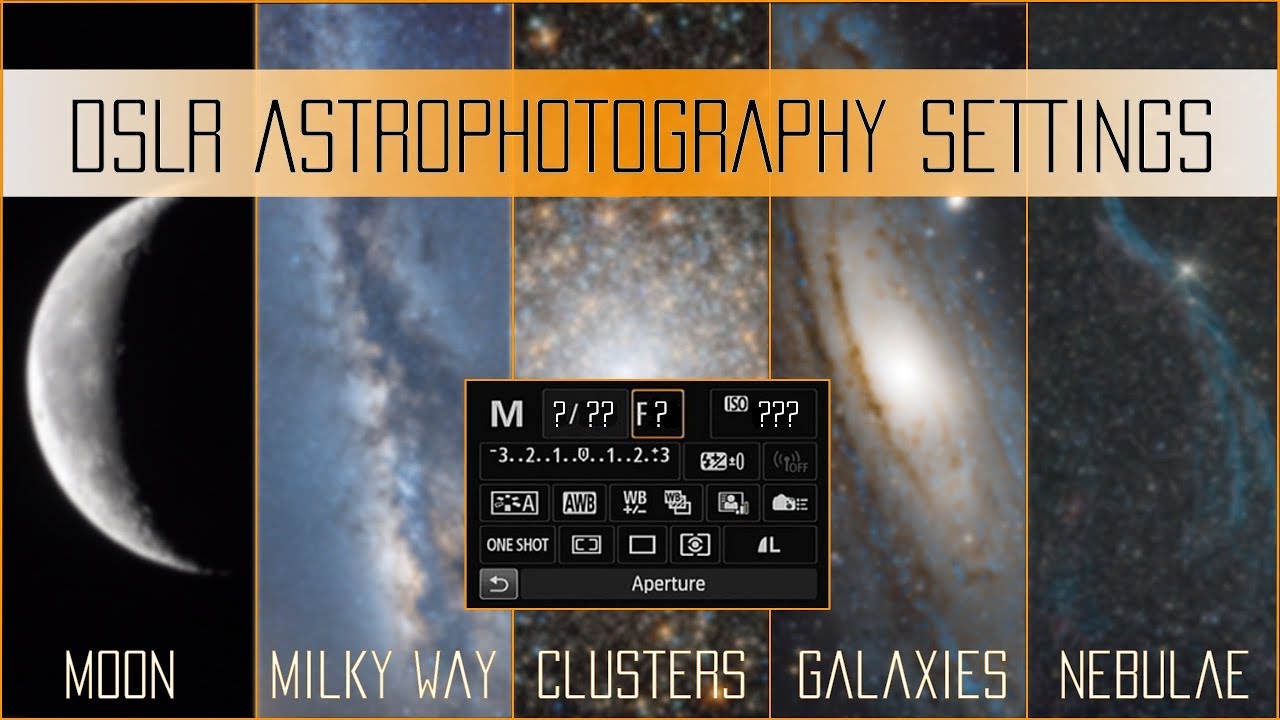This image displays an array of five photographs depicting various astronomical phenomena, including the Moon, the Milky Way, star clusters, galaxies, and a nebula. Each photograph is specifically labeled at the bottom with white text identifying the subjects as Moon, Milky Way, clusters, galaxies, and nebulae. Across the top of the image, a white and orange horizontal banner reads "DSLR Astrophotography Settings." Centrally located towards the bottom is a black rectangle showcasing camera or photo editing software settings. This section includes buttons and sliders for adjustments such as white balance, black levels, and aperture, with additional controls marked by numbers ranging from -3 to +3 and buttons adorned with question marks for further customization.